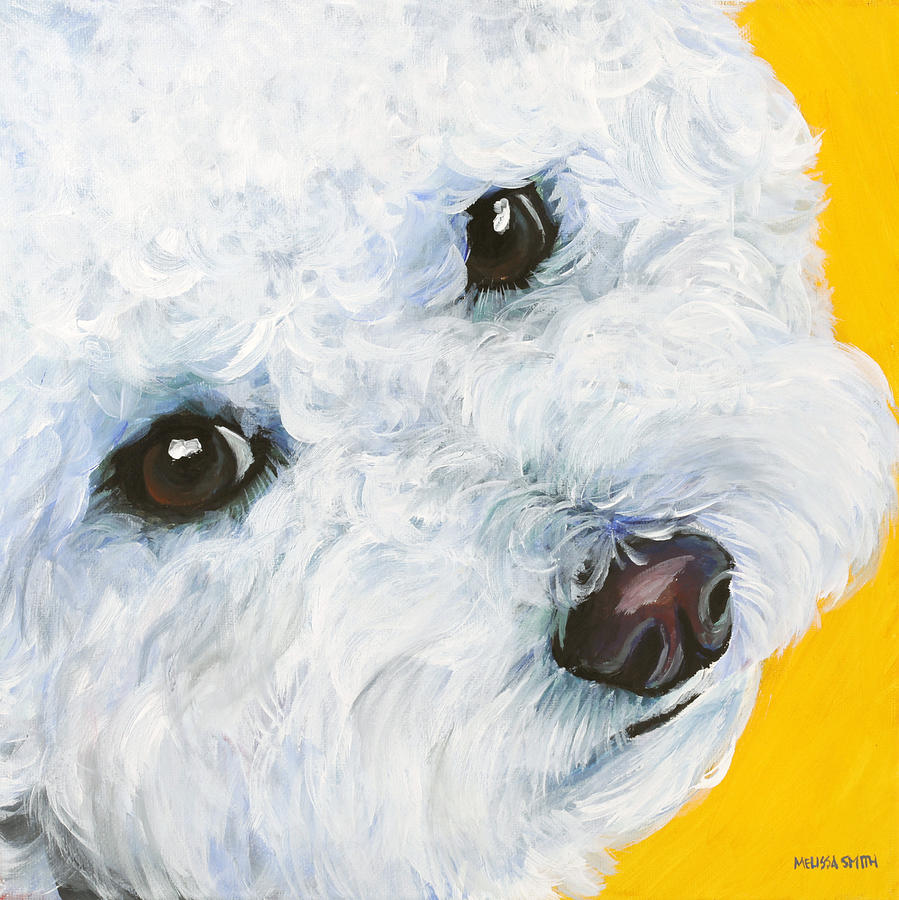This is an oil painting of a white poodle, with its face occupying almost the entire canvas. The poodle's short, curly fur appears predominantly white with subtle hints of blue or gray shading. Its large, brown eyes catch the light reflectively at the corners, and its nose is a soft brown with a hint of its black upper lip visible. The bright yellow background contrasts sharply with the dog's white fur. The artist, Melissa Smith, has signed her name in tiny letters in the lower right-hand corner of the painting.